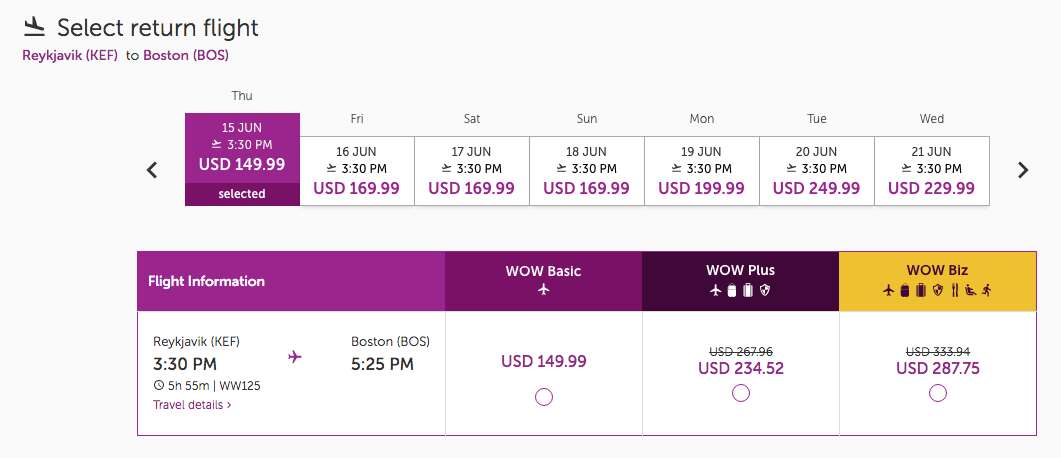This horizontal image showcases a flight selection interface, accessible via a computer website or a smart device through a website or app. The background is a flat, solid light gray without any texture or dimension. In the upper left corner, a black airplane icon is accompanied by the text "Select Return Flight." Below, in purple, the destinations Reykjavik (KEF) to Boston (BOS) are displayed.

A calendar interface is visible, highlighting Thursday, the 15th of June, with a selected time of 3:30 p.m. and a price of $149.99 USD. Additional options for other days of the week, from Friday through Wednesday, are shown with respective dates, times, and prices in USD.

Below the calendar, a horizontal bar provides detailed flight information: 
- Departure from Reykjavik (KEF) at 3:30 p.m.
- Flight duration of five hours and 55 minutes
- Landing in Boston (BOS) at 5:25 p.m.

The pricing tiers for the WOW airline are listed:
- WOW Basic: $149.99 USD
- WOW Plus: $230.52 USD
- WOW Biz: $287.75 USD